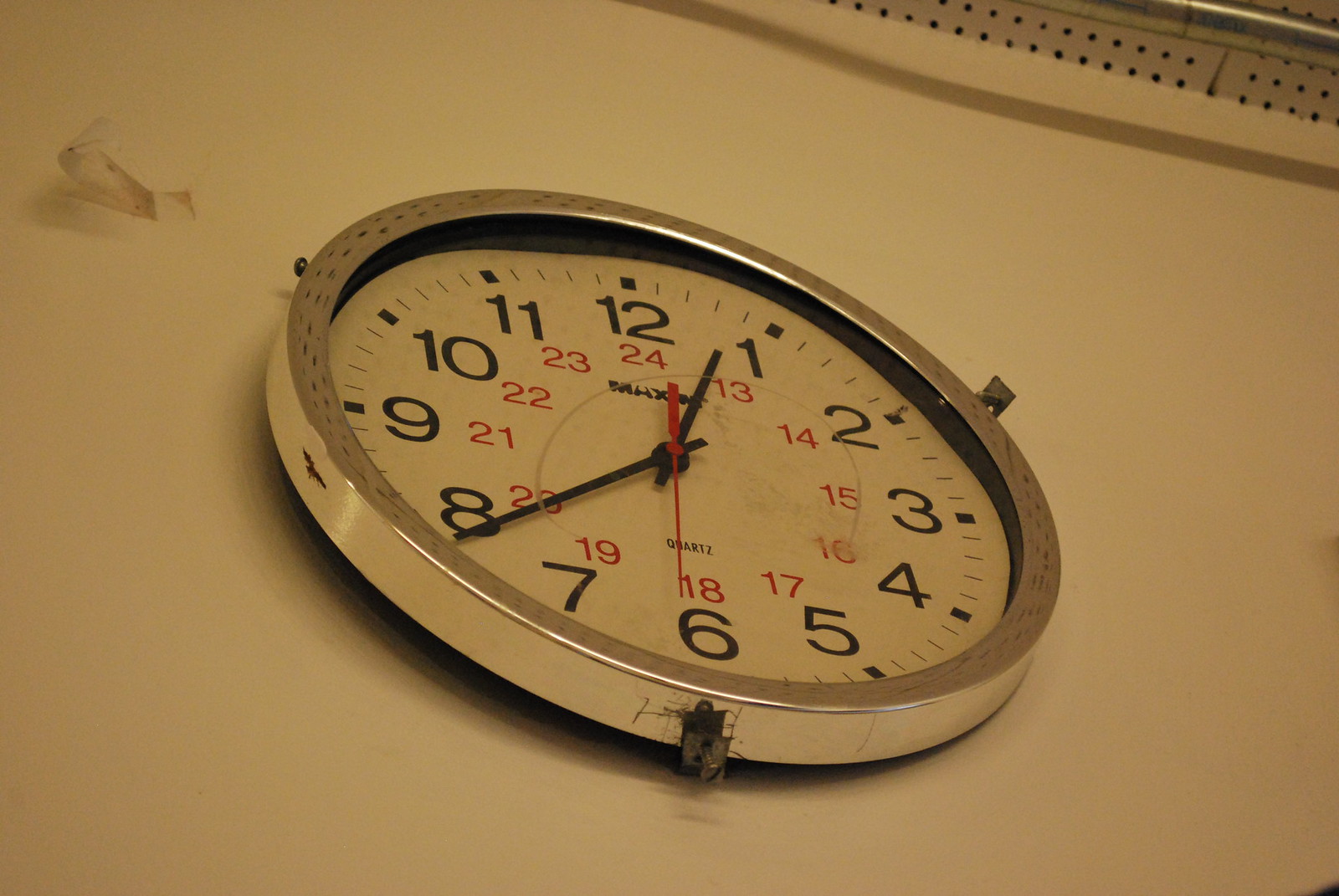The image depicts a round wall clock with a thick, reflective silver frame that might be chrome. The clock is mounted on a dull-colored wall. In the upper left-hand corner of the wall, there's an old piece of dirty tape, partially detached and curling outward. The clock's face is white, though it appears slightly warped and dirty, especially around the 16. The clock face is not covered by glass.

The clock showcases large black numbers arranged from 1 to 12 around the outer edge, with additional smaller red numbers from 13 to 24 indicating military time adjacent to the corresponding black numbers. The hour hand, minute hand, and second hand are all rectangular sticks, with the minute hand positioned between the 1 and the 12, and the second hand, a very thin red stick, positioned just past the 6.

Below the red number 18, the word "QUARTZ" is printed in small black text. The silver frame of the clock appears to have spots where it is cracked or worn, possibly around areas intended for mounting or hanging. In the background, towards the top right of the image, there is a white platform with a silver rod and some black holes, though their purpose is unclear.